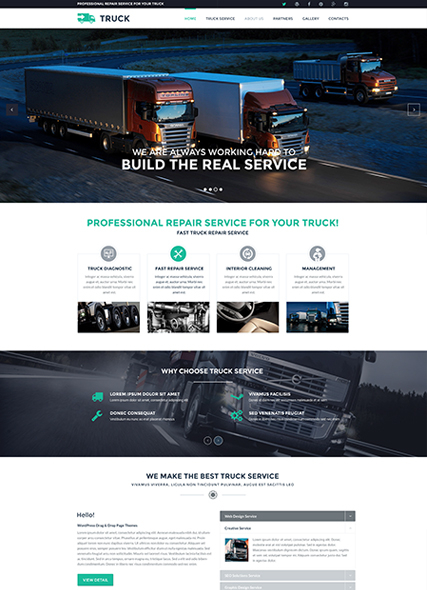**Caption:**

This screenshot showcases a trucking repair service website. At the top of the page, there's a small green truck icon accompanied by text that is too blurry to read. The main image features three trucks on a road at night: one appears to be a dump truck, while the other two are over-the-road trucks, like 18-wheelers. The over-the-road trucks are nearly side-by-side, with the dump truck positioned on the side of the road. 

Above the image, the text reads, "We are always working hard to build a real service." Below this, it states, "Professional repair service for your truck. Fast truck repair service."

The website offers four different services, each represented by icons, although the exact details are hard to decipher due to the blurriness. 

Further down, there's another banner featuring a truck captured head-on, driving down a road lined with trees. Text overlaying this image reads, "Why choose truck service," followed by four types of advantages, which are also blurry and difficult to read.

At the bottom of the page, the slogan, "We make the best truck service," is displayed. Additionally, there's a green button with text that is unfortunately too blurry to interpret, possibly prompting the user to view more details or services offered.